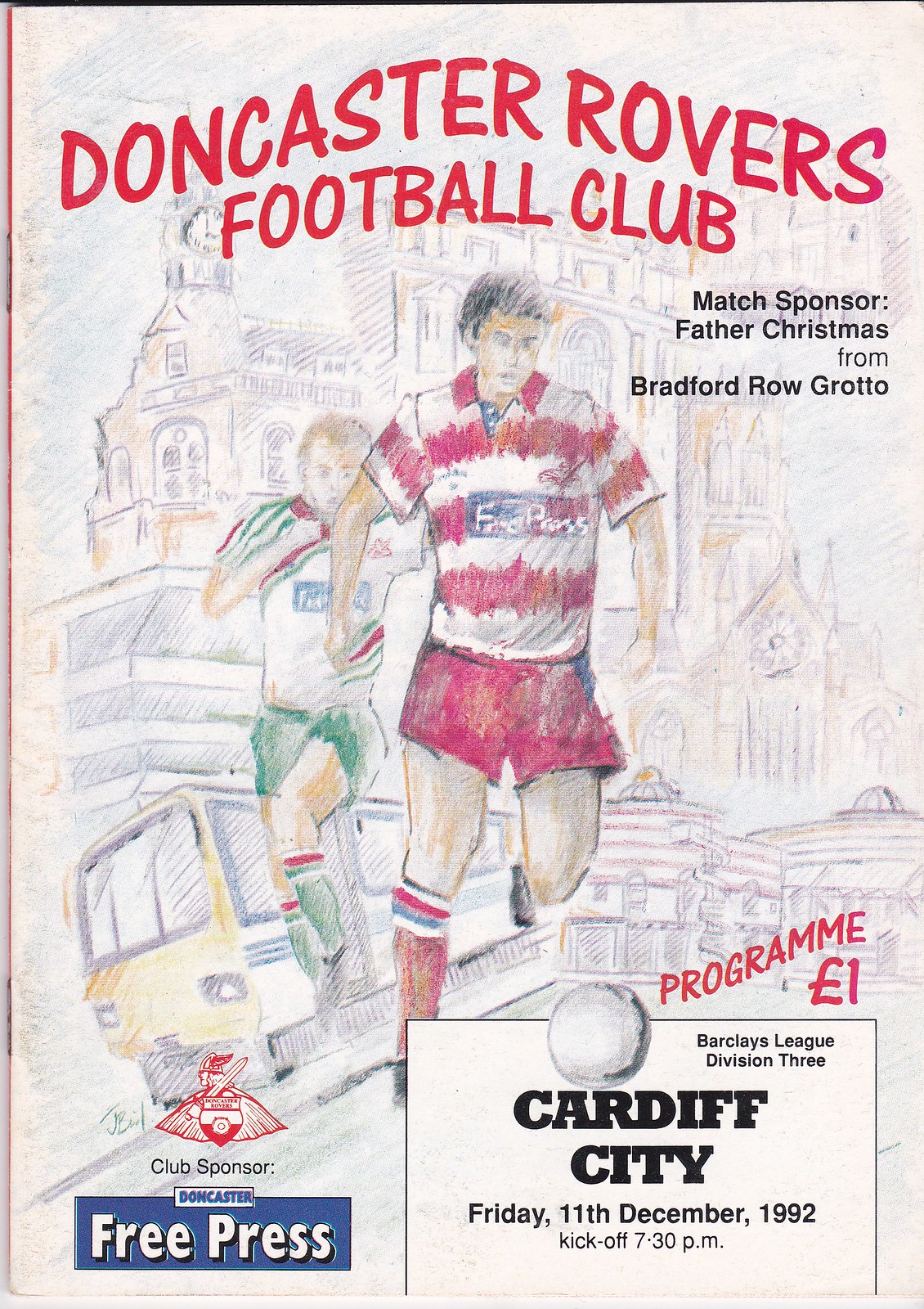This is a color photograph of the cover of a sports program for the Doncaster Rovers Football Club. The title is prominently displayed in red font at the top, with details indicating the match sponsor is Father Christmas from Bradford Row Grotto. Featured below is a pencil sketch of two young boys in sporting attire—one in a red and white striped jersey with red shorts and tall red socks, and the other in a green and white outfit with green shorts and tall green socks. The boy in the foreground, who appears larger, is poised to kick a white soccer ball, while the other chases behind him. The background includes a detailed city skyline with a train and a yellow city bus. Additional information includes the club sponsor, The Free Press, located at the bottom left, and the event details: Cardiff City, Friday, 11th December 1992, kickoff at 7.30pm. The word "PROGRAMME" is spelled out and the price is listed as one pound.